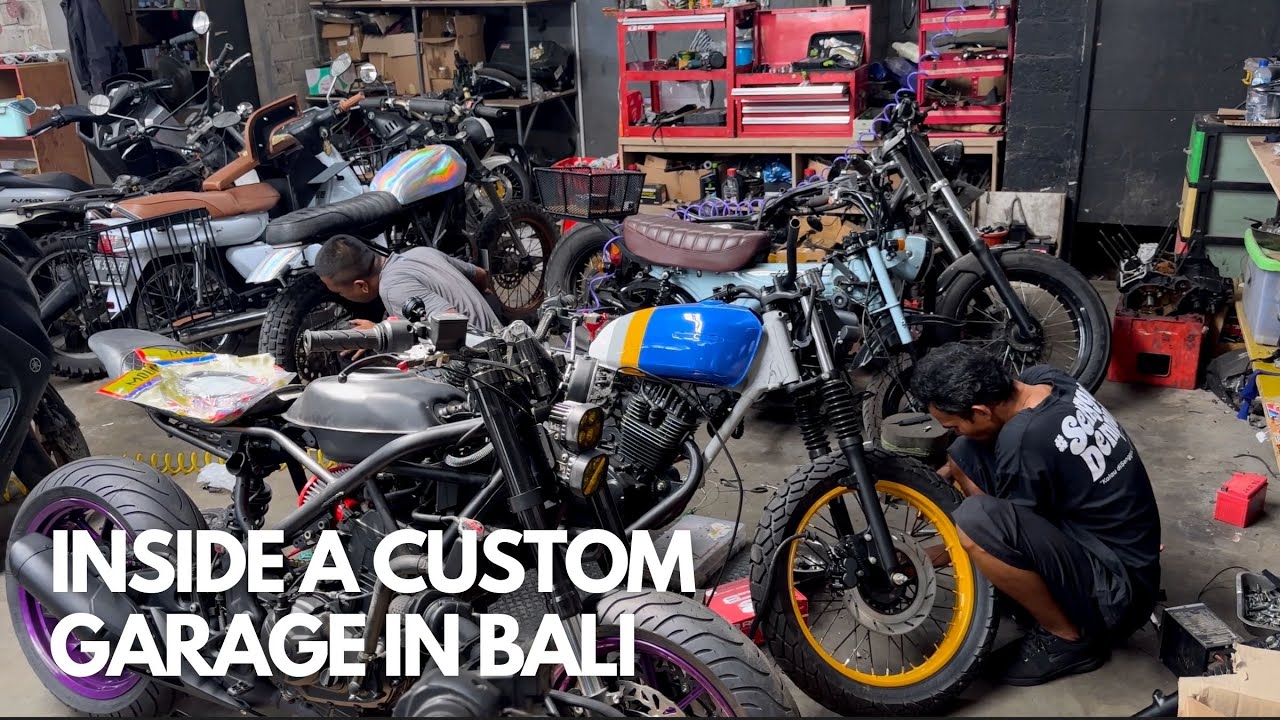Inside a custom motorcycle garage in Bali, the image captures a bustling, cluttered workspace filled with motorcycles in various stages of repair and customization. Dominating the scene, two mechanics are crouched on the ground, each diligently working on different bikes. The mechanic on the right, dressed in a black shirt and shorts, focuses on a predominantly black motorcycle featuring yellow accents around the front wheel. On the left, another mechanic wearing a gray shirt works on an all-black motorcycle. The shop itself is packed with at least nine or ten motorcycles, ranging from dirt bikes to other models, lined up along both sides. The background reveals a back wall adorned with black cupboards and red shelves, while a counter supports three large tool chests filled with tools and cluttered with various bike parts. Additional shelves and tool benches are scattered throughout, emphasizing the cramped and busy nature of this custom garage.